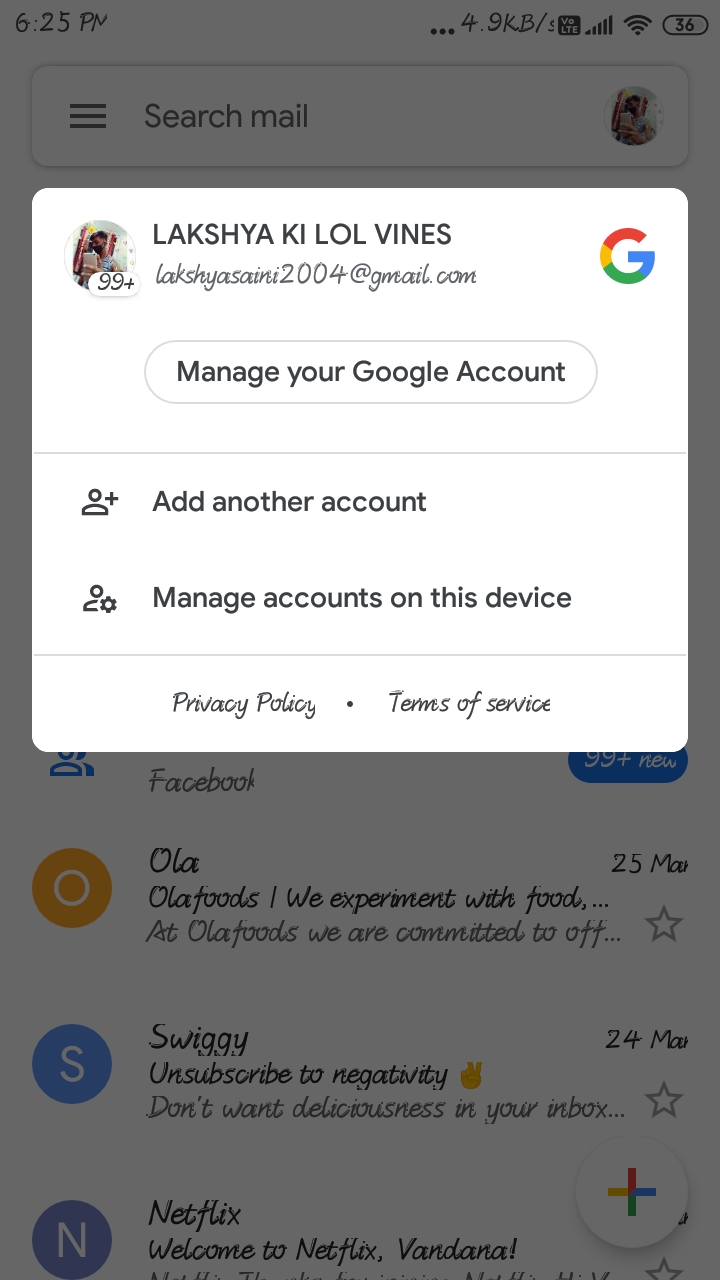The image showcases the settings page of a Gmail app on a smartphone. At the top of the screen, the status bar displays the current time, signal strength with several bars, and the Wi-Fi connectivity symbol. The main section prominently features a Gmail account, clearly identifiable by its email address. A button labeled "Manage your Google account" is situated at the top, providing access to account settings. Options to add another account or manage existing accounts on the device are also visible just below it. Further down, there are links to the privacy policy and terms of service.

The background of the image is filled with a list of emails from various companies such as Ola, Swiggy, and Netflix. These emails are displayed in black text against a white background. Each email is accompanied by a circular icon featuring the initial of the sender's name; for instance, Netflix emails are marked with a purple circle containing a white "N". The overall design maintains a clean look with predominantly white backgrounds and black text, typical of the Gmail application's user interface.